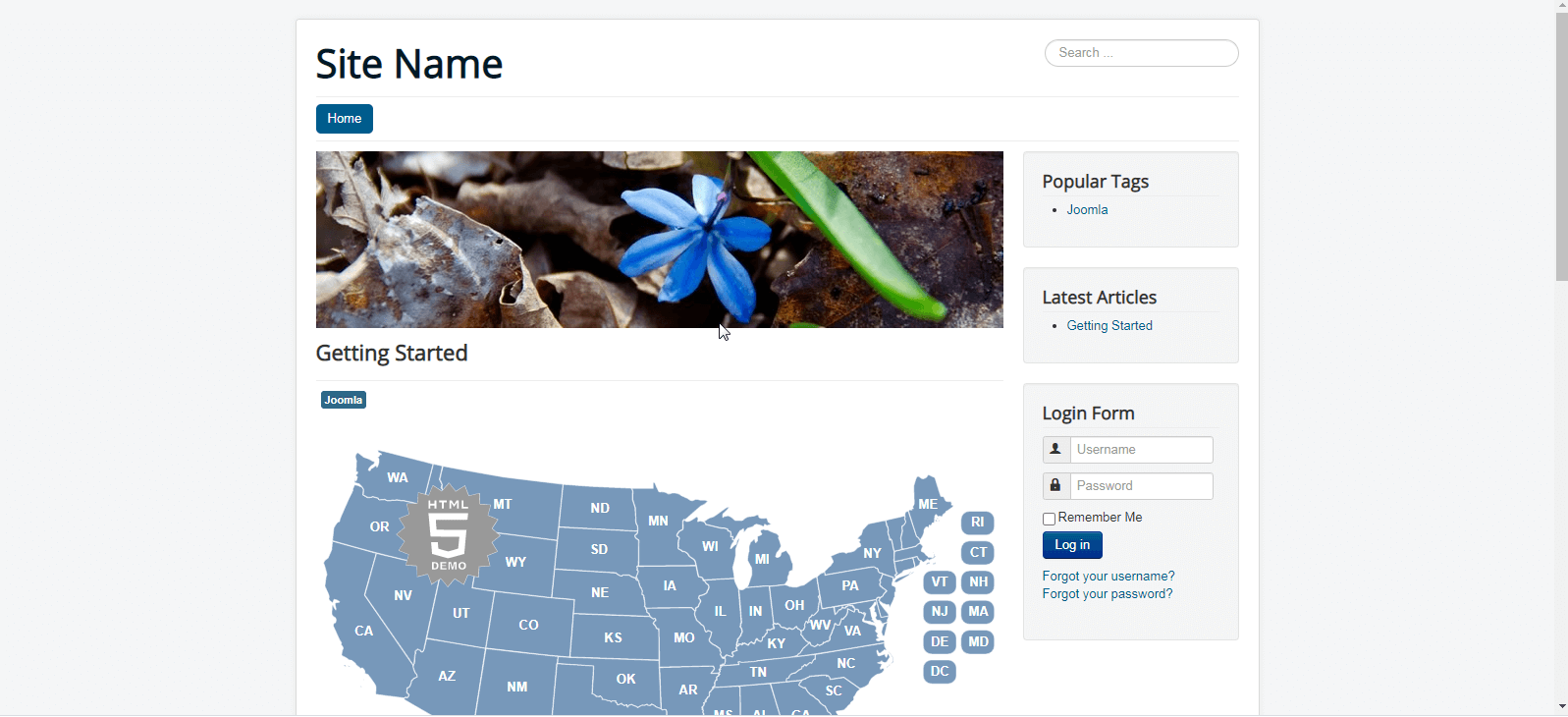The printout features a white background with a section titled "Site Name" at the top. To the right, there is an empty search bar. Below and extending from left to right, there is a blue, clickable tab with white text. Underneath this tab, there is a photo depicting a forested area featuring a blue flower and a partially visible green leaf.

To the right of the photo, there is a section labeled "Popular Tags" with the word "Jumia" highlighted in blue beneath it. Directly below the photo on the left-hand side, the words "Get Started" are written, with this section highlighted in blue. 

To the right of "Get Started," the words "Latest Articles" appear. Within the vicinity under the "Get Started" section, there is the word "Jumia" again in blue, accompanied by a map of the United States in blue with white state initials. 

A gray circle labeled "HTML5 Demo" is attached to the upper left side of the map. To the right of the map, there is a "Login Form" section containing fields for "Username" and "Password" along with clickable options for "Remember Me," "Login," "Forgot Your Username," and "Forgot Your Password."